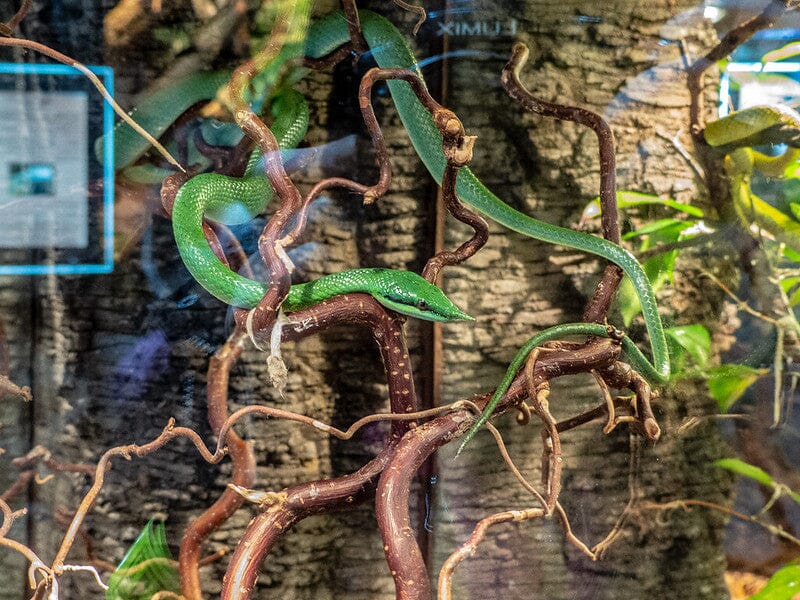This captivating photograph appears to be taken within a glass-enclosed snake exhibit at a zoo. The enclosure features an intricate setup with a winding vine, which may be real or artificial, and a few scattered leaves. Interwoven among the brown branches of what seems to be a tree, a vibrant green snake is visible. The snake, characterized by its distinctive reptilian skin and a tiny, keen eye on the right side of its head, appears to be at least two feet long and is elegantly coiled around the vines and branches. Soft hues of brown, green, black, and blue dominate the scene, complemented by reflections in the glass that suggest the glass barrier and hint at a framed picture in the top left corner and a brightly colored screen on the left side. The dual reflections confirm that the viewer is peering through a glass display, adding a layer of depth and realism to the detailed and serene image.